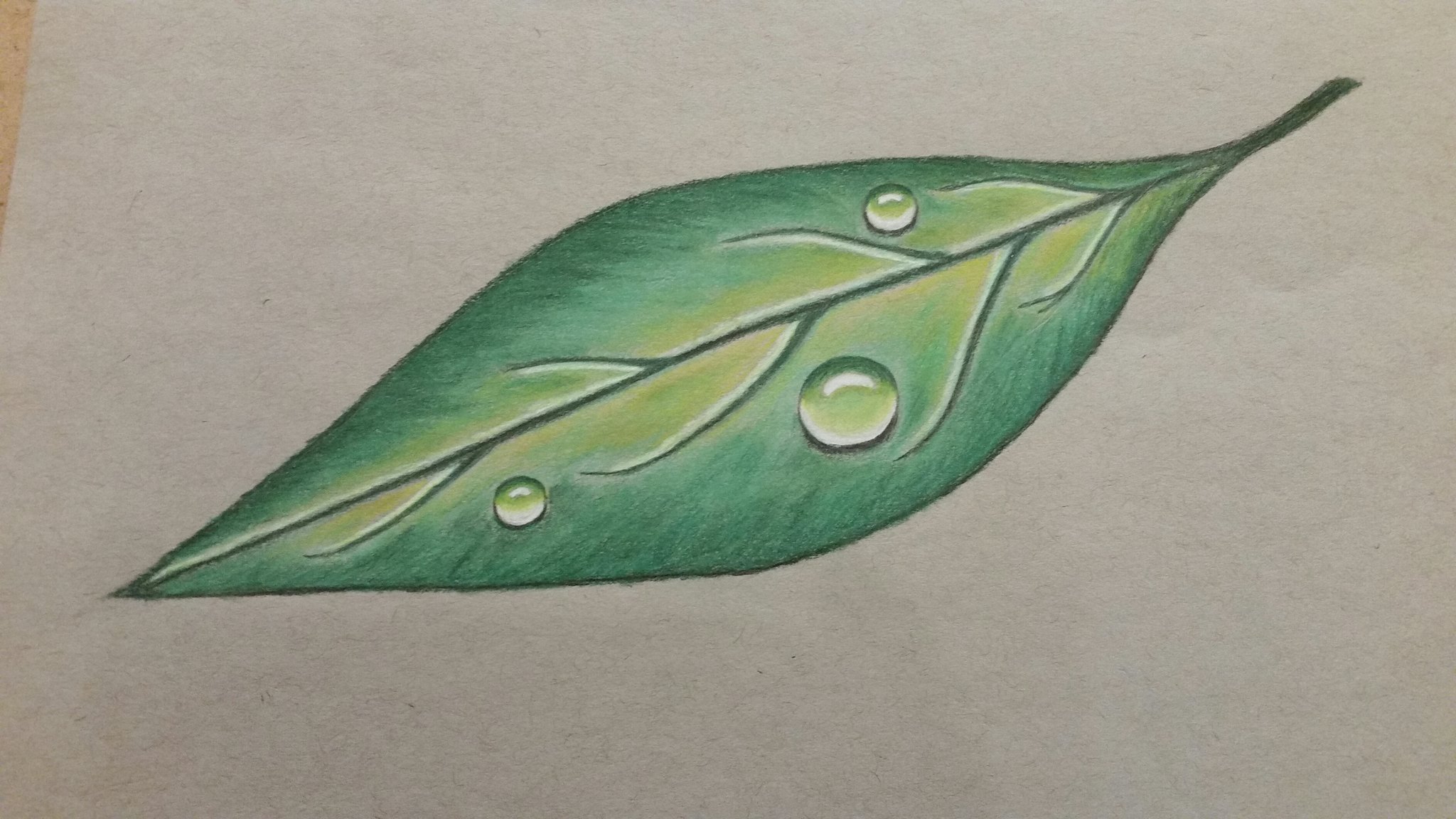The image features a meticulously detailed drawing of a single leaf, executed in colored pencil on a white piece of paper. The leaf is oval-shaped, tapering to sharp points at both ends, which makes its overall form resemble a human eye. The coloration is a rich gradient, with the outer edges being dark green, transitioning to medium green, and blending into a yellowish-green near the central vein. The central vein is dark green and runs down the middle of the leaf, from the stem positioned at the upper right to the point at the lower left, with several offshoot veins extending to the sides. Additionally, the leaf is adorned with three reflective water droplets, two positioned on one side of the leaf and one on the other, enhancing the realism of the drawing. The fine strokes and careful shading give the leaf a very lifelike appearance.